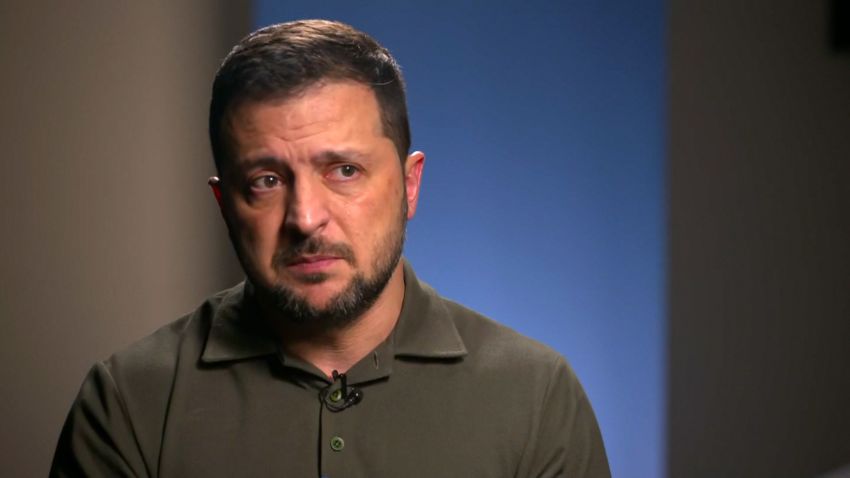The image depicts Volodymyr Zelensky, the President of Ukraine, positioned on the left-hand side of the frame. He is not looking into the camera but rather off to his left, suggesting he is engaged with someone else, likely an interviewer. His expression appears sad or concerned. Zelensky is dressed in a green button-up polo shirt, buttoned to the top, and he sports a beard and mustache. A microphone is clipped to the top of his shirt, indicating he is part of an interview or TV appearance. The background features a gray and blue striped pattern, illuminated by studio lighting that predominantly lights up his face. The colors in the image include shades of blue, muddy green, pink, black, and gray.